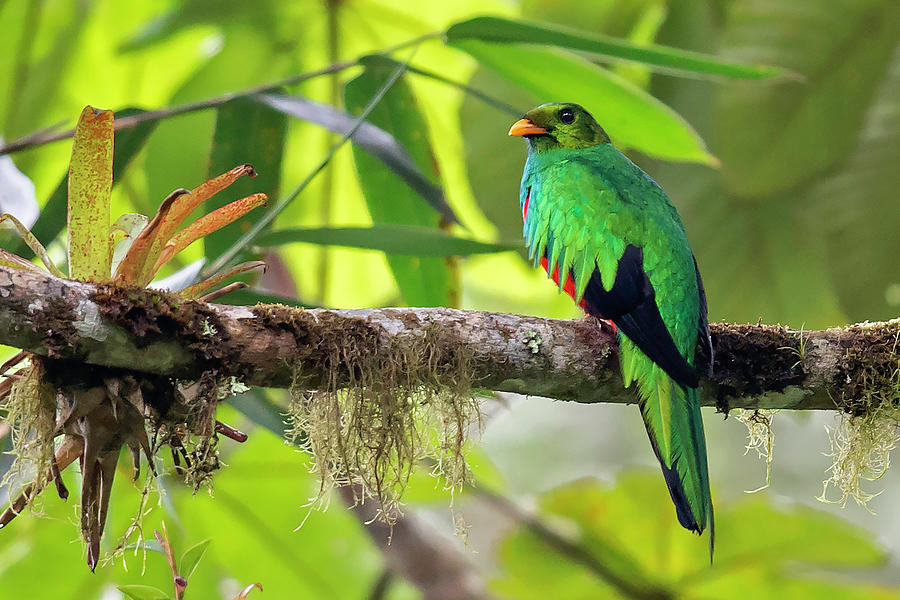This vibrant, high-quality photograph features a striking tropical bird perched on a moss-hung, horizontal tree branch within a lush jungle. The bird's back is a vibrant green, transitioning to dark navy blue or black feathers on its inner wings and tail. Its belly reveals a vivid apple red color, while its neck showcases patches of blue and red feathers. The bird's head is entirely green, sharply contrasted by its bright orange beak and piercing black eyes. The bird is positioned with its back to the camera, its head turned slightly towards the lens. Surrounding the branch are large, banana-like leaves and other dense foliage, evoking the atmosphere of a thriving rainforest. The image is clearly taken during daylight, highlighting the natural habitat of this exotic avian species.